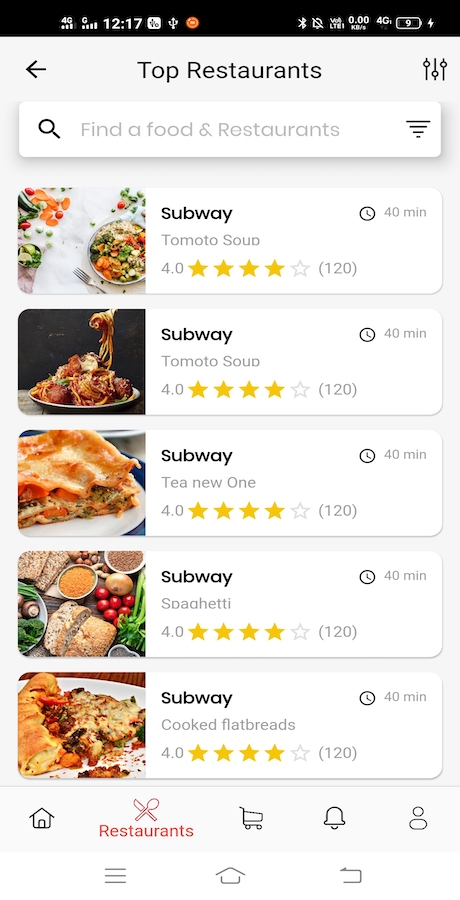Screenshot Description:

The top section of the screenshot features a black bar with various white icons indicating device status. From left to right, you can see a 4G symbol for network status, a time display showing 12:17, what appears to be a signal strength icon resembling a white pitchfork, an orange notification icon, a Bluetooth symbol, and a battery icon.

Beneath the status bar, there is a navigation section. It includes a black back arrow on the left and the text "Blacktop Restaurants." This is followed by a white search box containing a black magnifying glass icon and a funnel icon, likely for filter options.

Below the navigation, the main content area presents a selection of dishes from a restaurant. The first dish listed is labeled "Subway Tomato Soup," accompanied by an image of salad and vegetables on a white surface. The dish details show a preparation time of 40 minutes, a rating of 4 stars, and a total of 120 reviews.

The next image depicts spaghetti and meatballs with the same "Subway Tomato Soup" label, 40-minute preparation time, 4-star rating, and 120 reviews.

Following this, there is an image of a tan, flaky Italian dish garnished with pesto, labeled "Subway Tea." It maintains the same details: 4-star rating, 120 reviews, and a 40-minute preparation time.

The fourth dish is "Subway Spaghetti," also rated 4 stars with 120 reviews and a 40-minute prep time. This image showcases a mix of red and green vegetables, along with bread.

Concluding the dishes section is "Subway Cooked Flatbreads," displaying an Italian pasta dish. The details again reflect a 4-star rating, 120 reviews, and 40 minutes to prepare.

At the bottom of the screenshot, a gray house icon is seen next to a red spoon and knife icon labeled "Restaurants." Additionally, there are icons for a card, a bell, and people. Further down, there are repeated icons for a house and a back arrow.